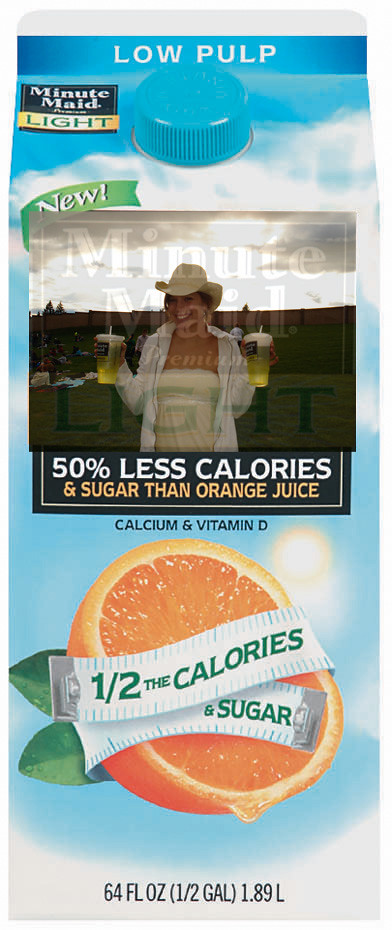This image features a 64 fluid ounce (1.89 liter) carton of Minute Maid Light Orange Juice, prominently showcasing the front label. The carton is primarily printed in blue and white, with a notably blue plastic spout at the top. On the label, an illustration of an orange sliced in half is present, alongside a tape measure banner that proclaims "Half the calories and sugar." 

Additionally, there is a boxed-in section featuring a photograph of a woman grinning widely. She is holding two plastic cups with lids and straws, each containing an amber-colored transparent liquid. The woman is attired in a white halter top paired with a shirt and a cowboy hat. Beneath her image, text reads: "50% less calories and sugar than orange juice, calcium and vitamin D."